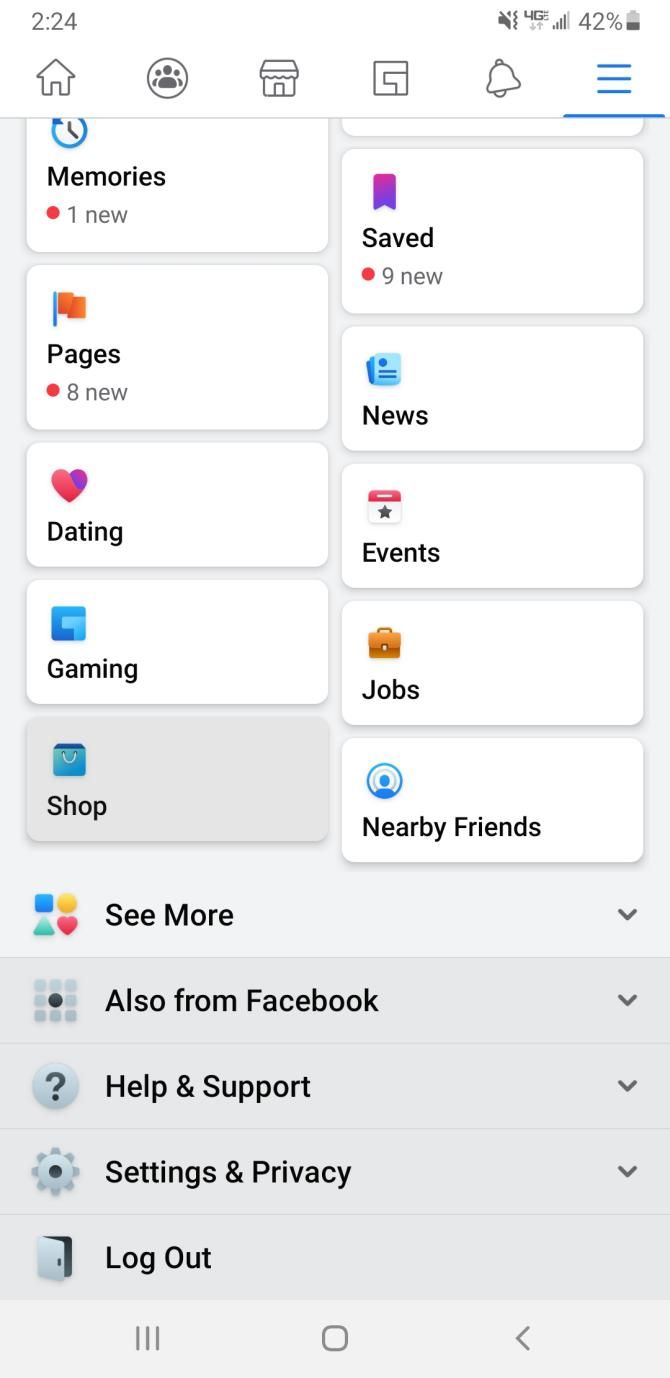This screenshot from a mobile phone displays various interface elements, providing insightful details about the device's status and available features. At the very top, a white status bar shows the current time as "2:24" in a gray font on the upper left corner. On the upper right corner, icons indicate a muted microphone, "4G LTE" network connectivity, a mobile signal strength, "42%" battery life, and a corresponding battery icon.

Following the status bar, there is a navigation bar with five distinct icons: a home icon resembling a house, a circle with three people symbolizing social connections, a storefront icon for marketplace access, a prominent 'G' icon possibly related to Google, and a bell icon for notifications.

Below the navigation bar, a section of white rectangles organizes different sections of the mobile phone's interface. On the top left, there is a "Memories" section accompanied by a clock icon, indicating "1 new" update. Beneath that, a "Pages" section with a flag icon shows "8 new" updates. The subsequent sections include "Dating" (heart icon), "Gaming" (G icon), and a grayed-out "Shop" (shopping bag icon).

On the top right, a "Saved" section with a bookmark icon indicates "9 new" items. Below it, a "News" section marked by a newspaper icon appears to provide access to recent news articles or updates.

This detailed interface layout highlights the phone's functional areas, providing a comprehensive overview of the user’s available tools and current notifications.